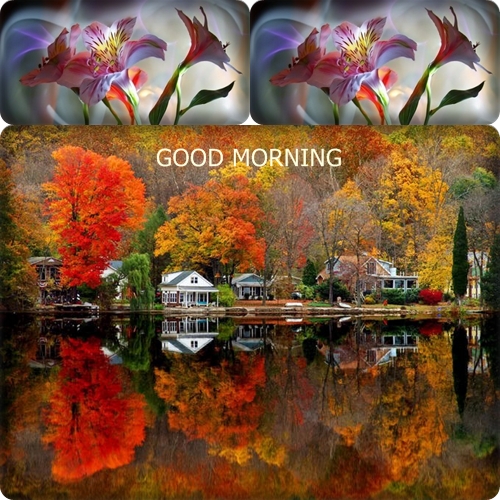The image is a vibrant fall scene, segmented into three distinct parts. The bottom, and main section, features a tranquil lake with a stunning mirror-like reflection of the surrounding scenery. Along the lake’s shore, there are several small houses or cottages, painted in various colors including white, dark blue, and brown. These houses are partially obscured by a dense array of trees showcasing a breathtaking autumn palette of fiery oranges, bright reds, sunny yellows, and some lingering greens, with a few trees already bare.

The top portion of the image is divided into two smaller, square photographs. Each of these squares contains a close-up of vibrant pink flowers with green stems; the flowers are presented against a graphic design background featuring elements resembling electricity and bubble patterns in white.

Overlaying the main photograph of the lake and cottages, written in all capital letters in a light beige font, is the cheerful greeting: "GOOD MORNING." This text stands out against the vivid fall landscape, harmonizing with the vibrant and serene atmosphere of the scene.